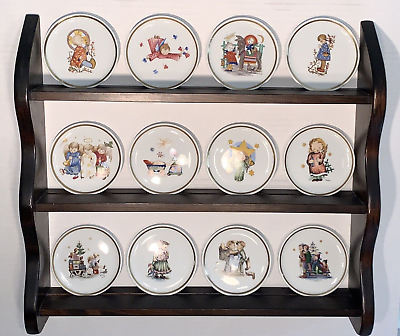A photograph displays the upper shelving portion of a vintage hutch, likely from the 50s or 60s, made of dark walnut wood with scalloped edges. This hutch stands against a white wall and features three rows of shelves, each hosting four small, decorative plates, totaling twelve. The plates, which seem to be part of a curated collection by the same maker, have a dark charcoal rim and showcase a variety of intricate, old-fashioned art designs. The artwork includes figurines and animals, with recurring themes of children, Christmas imagery such as Christmas trees and presents, and even a childlike angel with a halo. The images are drawn in a style reminiscent of Thomas Kinkade, incorporating light, colorful palettes with shades of red, tan, gray, blue, brown, gold, and green. The light reflects softly off the shiny surfaces of the plates, enhancing their detailed, whimsical illustrations.